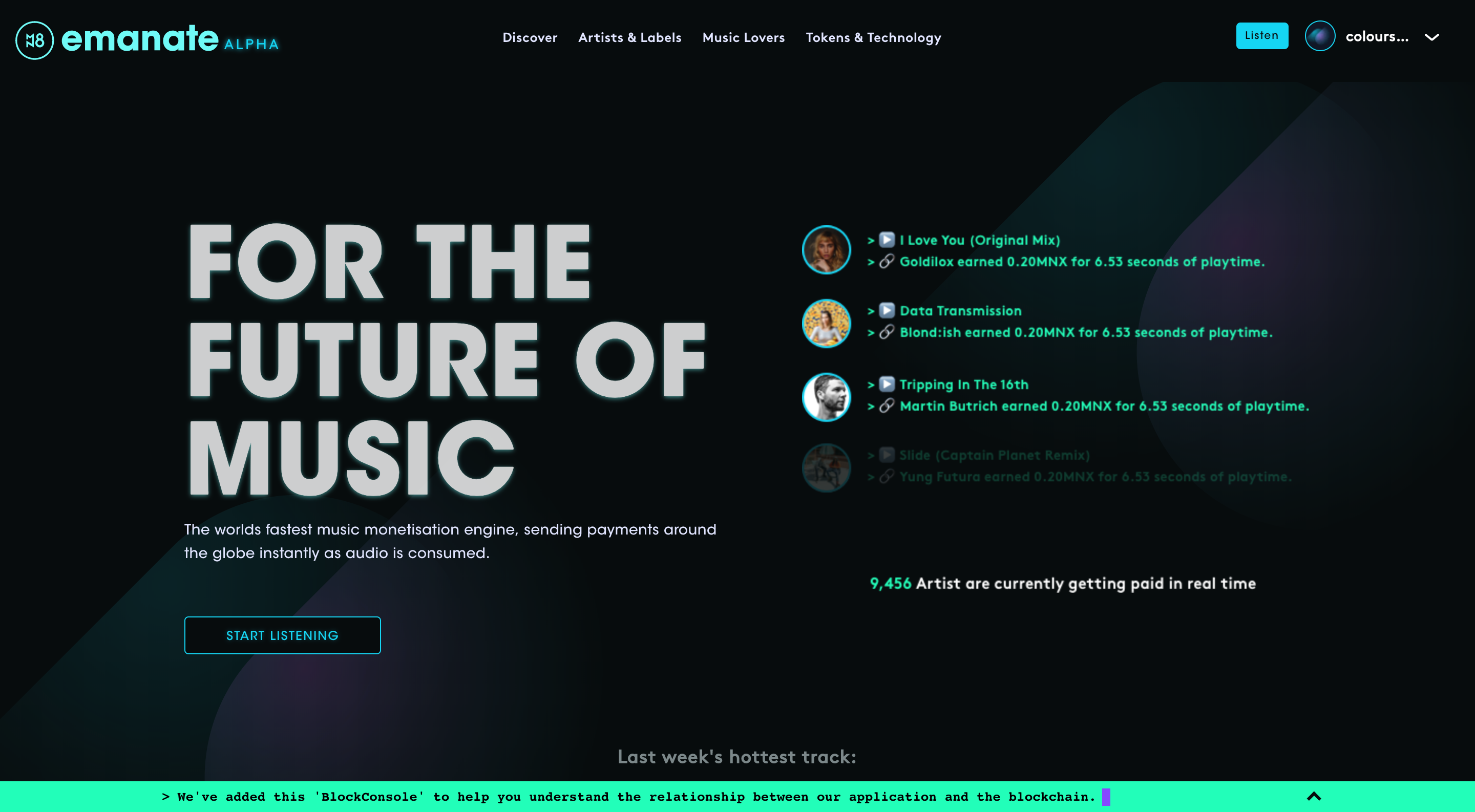This is a screenshot from the Emanate Alpha website, showcasing its sleek and modern design. The background is black, featuring subtly faded, amorphous shapes in green and purple hues that highlight the crispness of the foreground text. At the top, a navigation menu includes options like "Discover," "Artists and Labels," "Music Lover," and "Tokens and Technology." A prominent blue button with black text invites users to "Listen," while a nearby dropdown menu labeled "Colors" suggests a user control panel, though the text is partially cut off.

A large header boldly declares, "For the Future of Music," followed by a subheading touting Emanate as "The world's fastest music monetization engine, sending payments around the globe instantly as audio is consumed." Beneath this, a black button with blue text offers a call-to-action to "Start Listening."

To the right of this section, various icons and links likely represent different songs and possibly information about earnings, with an emphasis on current top earners. It's noted that "9,456 artists are currently getting paid in real time."

At the bottom of the screen, a partially visible text snippet reads "Last week's hottest track." Additionally, a popup bar with an aqua background and black text provides users with insights into the relationship between the application and blockchain technology, displayed as a thin line at the bottom of the page.